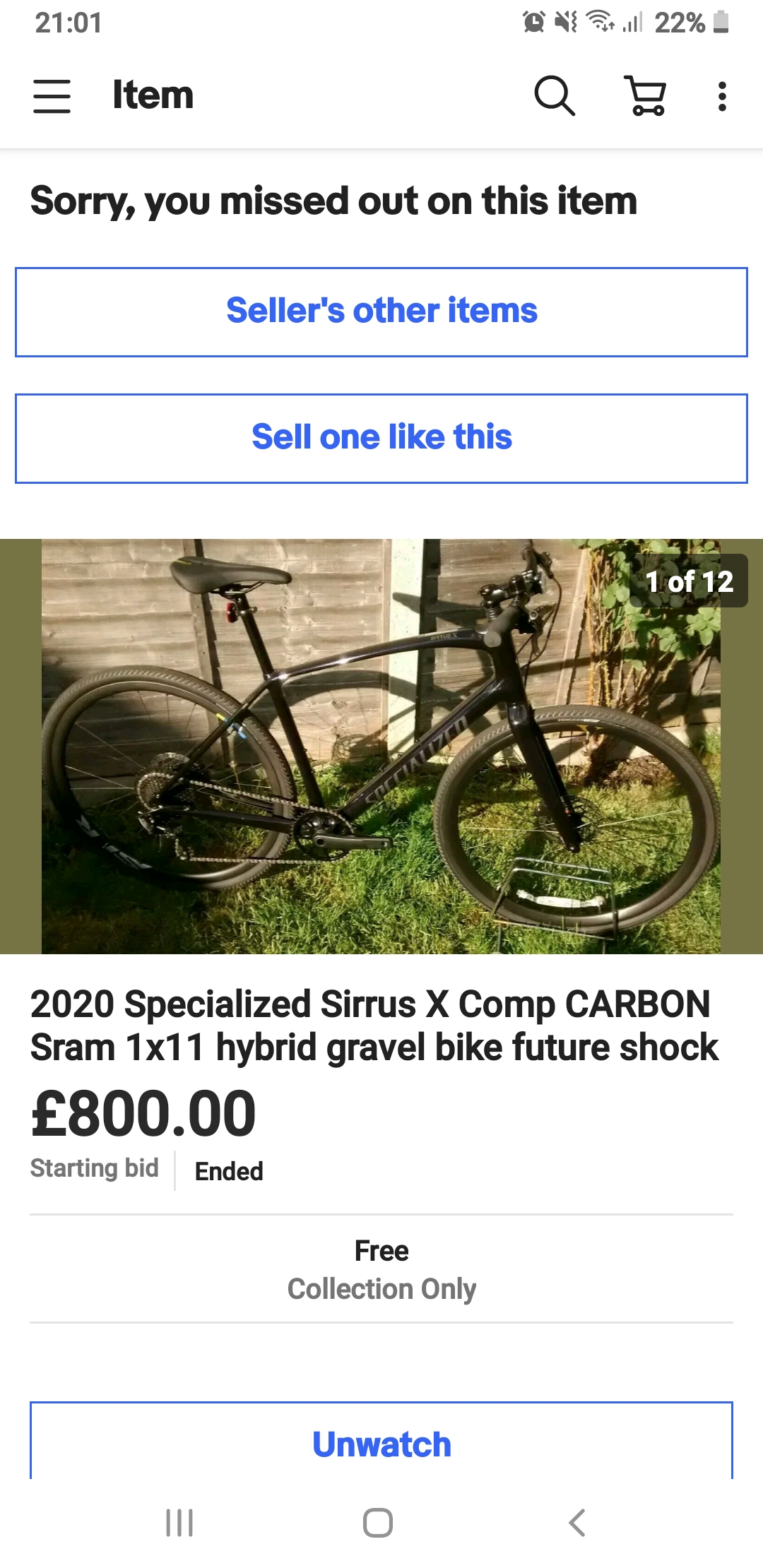**Descriptive Caption:**

A smartphone screenshot reveals an active auction on a marketplace app. At the top, the timestamp reads "21:01." To the right of this, an alarm icon, sound icon (muted), Wi-Fi icon, and battery indicator (at 22%) are visible. Below this header, the interface features a hamburger menu on the left, followed by a search icon, a shopping cart, and a menu with three vertical dots.

The main body of the screenshot contains a message that says, "Sorry, you missed out on this item." Below this notice are two sections: "Seller's other items" and “Sell one like this.”

The image features a bicycle photograph labeled "1 of 12." The bike is black and appears to be a lightweight, racing mountain bike. Further details reveal it is a "2020 Specialized Sirrus X Carbon SRAM 1x11 Hybrid Gravel Bike with Future Shock." The starting bid is listed at 800 euros and the auction has been extended. It's noted that the bike is available for "Free collection only."

At the bottom of the screen, there’s a prompt showing "Unwatch" (indicating the option to remove the item from the watchlist), a button symbolized by a downward arrow to navigate further down the page, a home button, and a left-facing arrow for going back to the previous page.